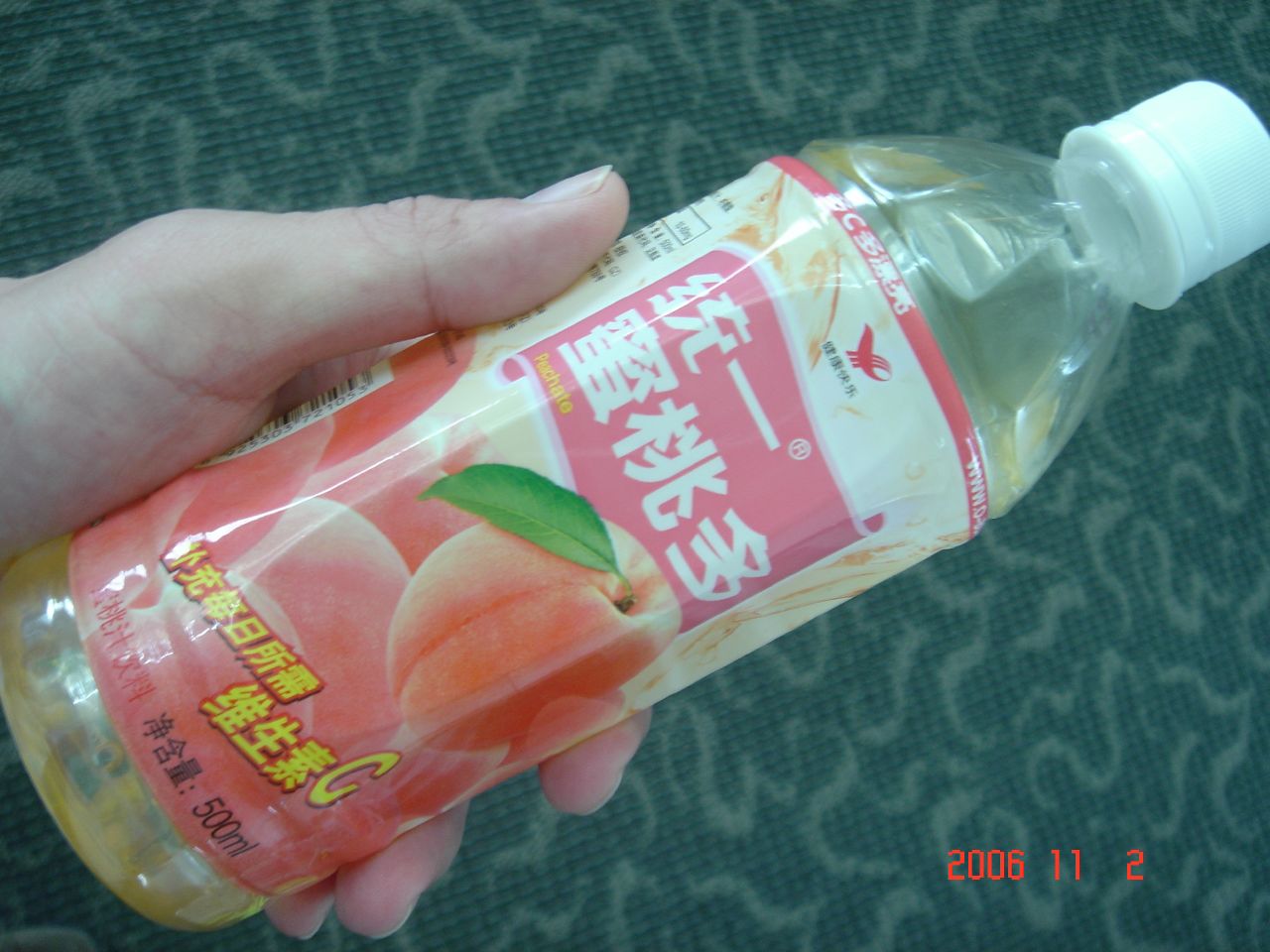A hand holds a horizontally positioned juice bottle, angled diagonally from the bottom left to the top right of the image. The backdrop reveals a greenish carpet with a wavy line pattern. The juice bottle, likely containing apple juice, appears to be a Japanese brand given the Japanese text on the label. The liquid inside has the characteristic amber hue of apple juice, and the label features vibrant imagery of apples. At the bottom, the label is predominantly red with a cluster of apple illustrations, while the top part is white, showcasing a red banner with the brand name written in Japanese characters. The bottle is capped with a white lid and has a slight dent near the top, giving it a slightly worn appearance.